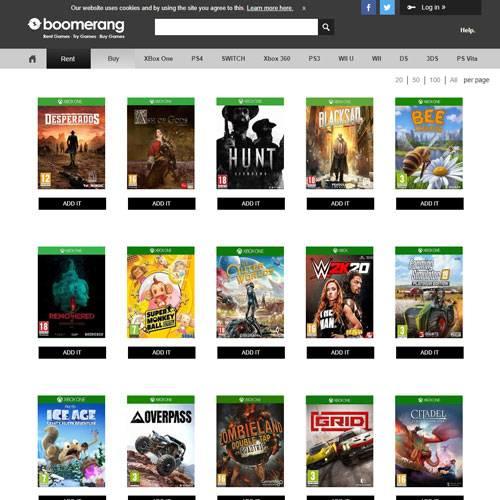This is a detailed screenshot of a computer screen displaying a video game rental and purchase website interface. The central portion of the screen showcases a grid matrix of 15 video game cover images organized in a format of five columns by three rows. These games predominantly appear to be for the Xbox platform, though this isn't explicitly confirmed.

At the top of the screenshot, there's a navigation bar. In the upper left corner, the word "Boomerang" is displayed in white text, suggesting the name of the website or application. Adjacent to it is a white search bar, accompanied by a magnifying glass icon on its right side for search functionality.

Below this navigation bar is another horizontal grey bar containing interactive tabs. The "Home" tab appears first, followed by the "Rent" tab, which is highlighted in black, indicating it is currently selected. Moving further right, there are several tabs, each labeled with different gaming platforms, including Xbox One, PS4, Nintendo Switch, Xbox 360, PS3, Wii U, Wii, DS, 3DS, and PS Vita, implying that users can navigate through various video games categorized by these systems.

In summary, the screenshot depicts an organized and user-friendly interface from a video game rental and purchase website, mainly displaying Xbox games, and provides multiple search and navigation options.